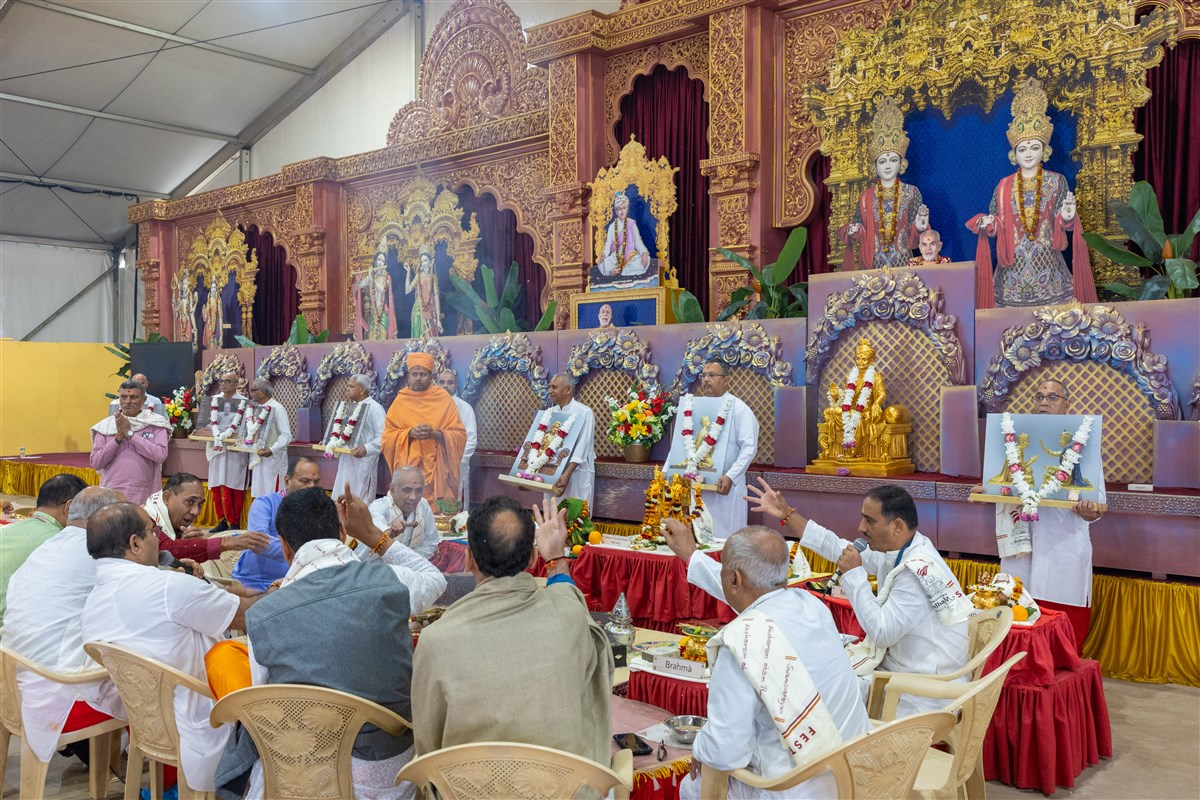This color photograph captures a detailed scene of a Hindu religious ceremony. In the foreground, approximately nine men are seated at a long table. Many of them have one hand raised in the air, suggesting they are participating in a ritual. Lined behind these men are about six others dressed in white robes, holding garlands. Among them, a person stands out adorned in a vibrant orange robe and cap. The background is striking with an ornate platform displaying statues of Hindu gods and goddesses, richly adorned in red, orange, yellow, and gold. The platform itself is predominantly light red with intricate gold ornamentation. The setting is clearly religious, marked by the symbolic use of colors and the presence of arches embellished with gold and royal blue accents. The men in white robes exude a sense of holiness, contributing to the spiritual atmosphere of the ceremony.